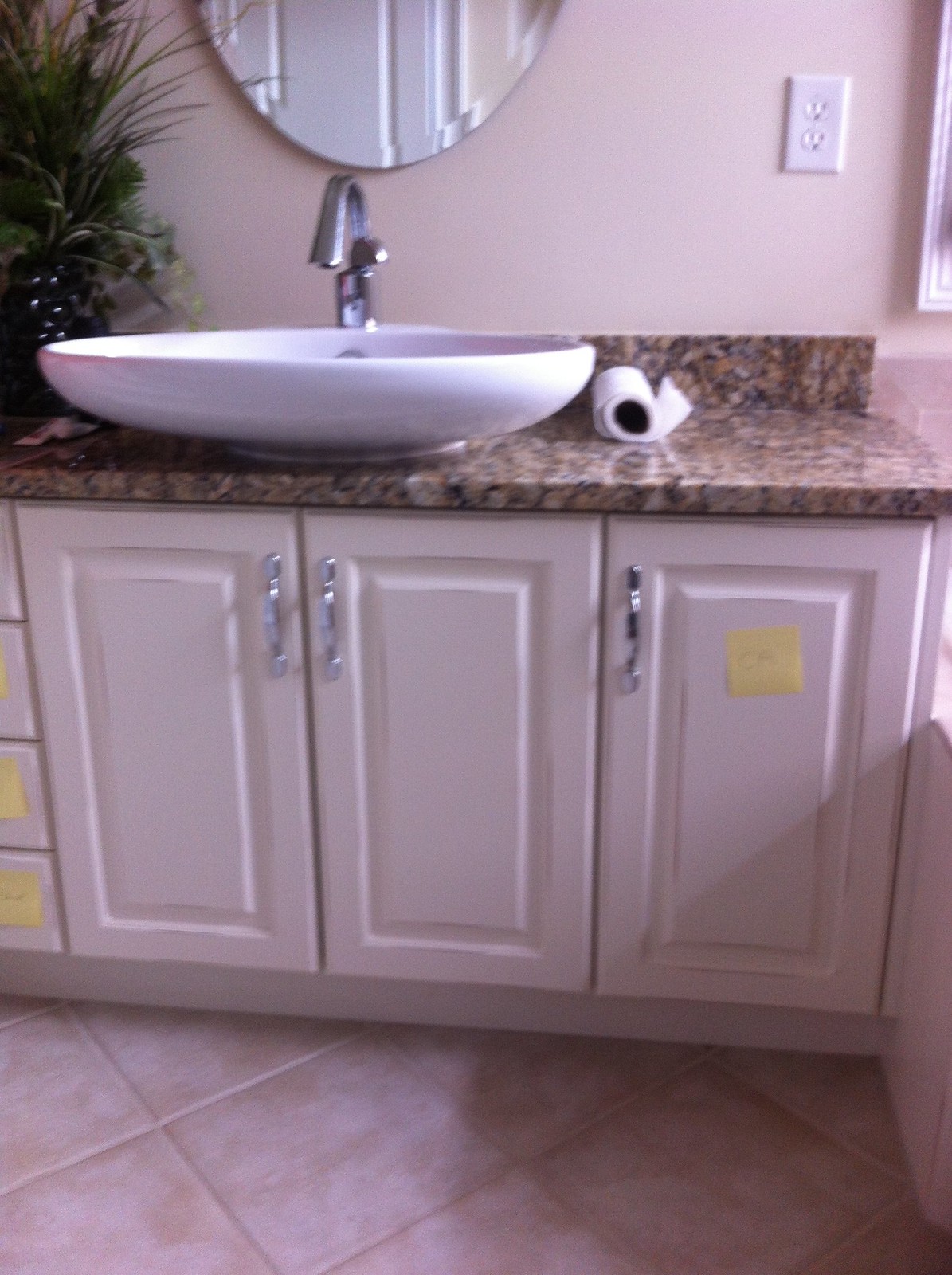A detailed photo of a bathroom features diamond-shaped, creamy off-white and beige tiles, with darker beige areas likely due to shadows. The bathroom includes a granite countertop, showcasing a mix of brown hues and a hint of yellow. On the countertop, there's a nearly depleted roll of toilet paper. A white bowl sink rests atop the counter, adorned with silver hardware. Just above the sink, the edge of a white-rimmed mirror is visible. To the left of the sink, a green potted plant adds a touch of nature. Below the countertop, there are cabinets including one section with four drawers, each labeled with yellow sticky notes. Adjacent to these drawers are two cabinet doors, and to the right, another single cabinet door also marked with a sticky note. The walls of the bathroom are painted in an off-white color.